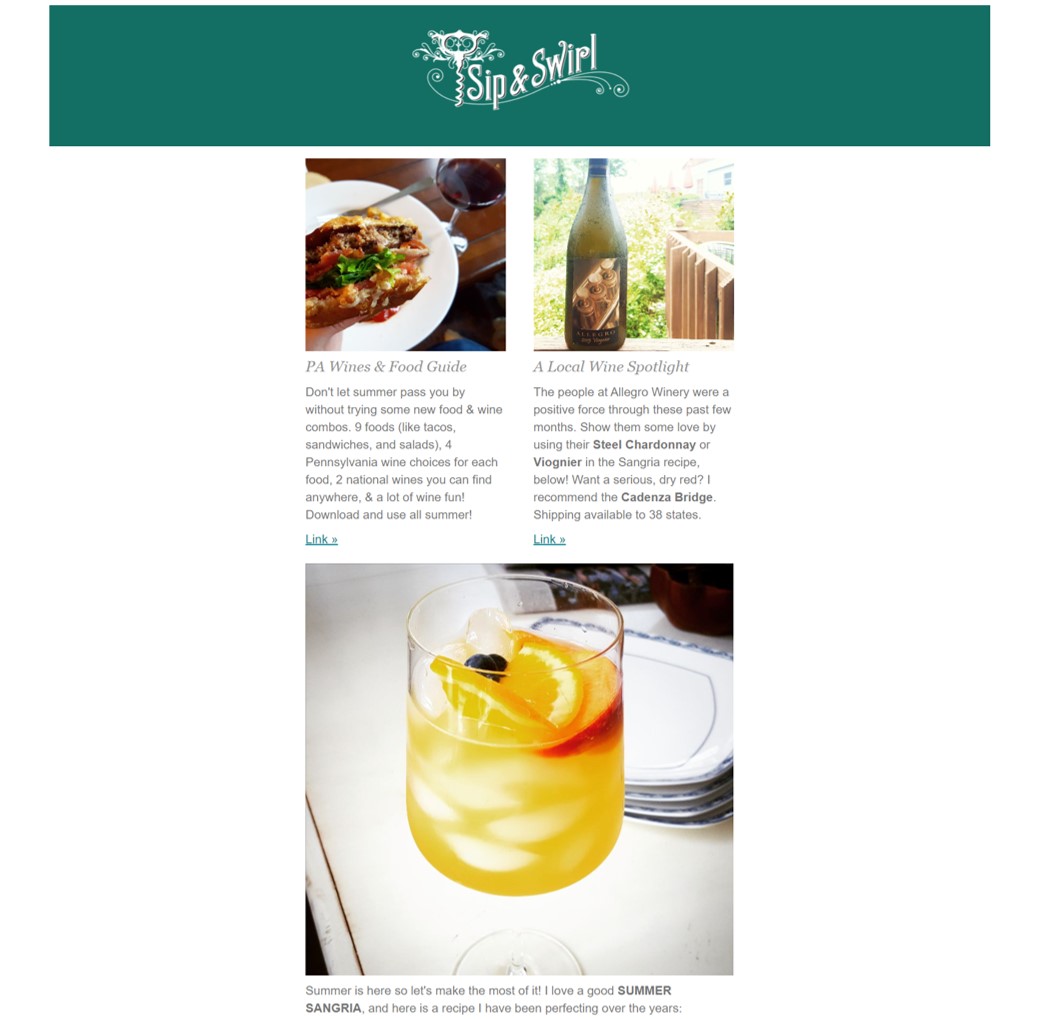At the top of the image, a cool green banner extends from left to right, featuring the phrase "Sip and Swirl" in elegant white font, centered with a flourishing curve. To the left of "Sip," a wine opener corkscrew tool adds a touch of sophistication. 

Beneath the banner, the image is divided into two main sections. On the left, there's a box showcasing a white dish with tantalizing food, including what appears to be chicken and lettuce, accompanied by a wine glass filled with rich red wine. Below this, the text in grey font reads:

"PA Wines and Food Guide

Don't let summer pass you by without trying some new food and wine combos. Nine foods, like taco sandwiches and salads. Four Pennsylvania wine choices for each food. Two national wines you can find anywhere, and a lot of wine fun. Download and use all summer."

A light blue hyperlink labeled "Link" is situated beneath this text.

To the right of this box, an image displays a green wine bottle with the subtitle "A Local Wine Spotlight." Below the bottle, the description reads:

"The people at Allegro Winery were a positive force through these past few months. Show them some love by using our Steel Chardonnay or Visioneer in the sangria recipe below. Want the series dry red? I recommend the Cadenza Bridge. Shipping available to 38 states."

Another hyperlink labeled "Link" is positioned below this text.

At the bottom of the image, a final box features a picture of a vibrant yellow margarita garnished with orange slices, adding a splash of summer zest to the overall design.